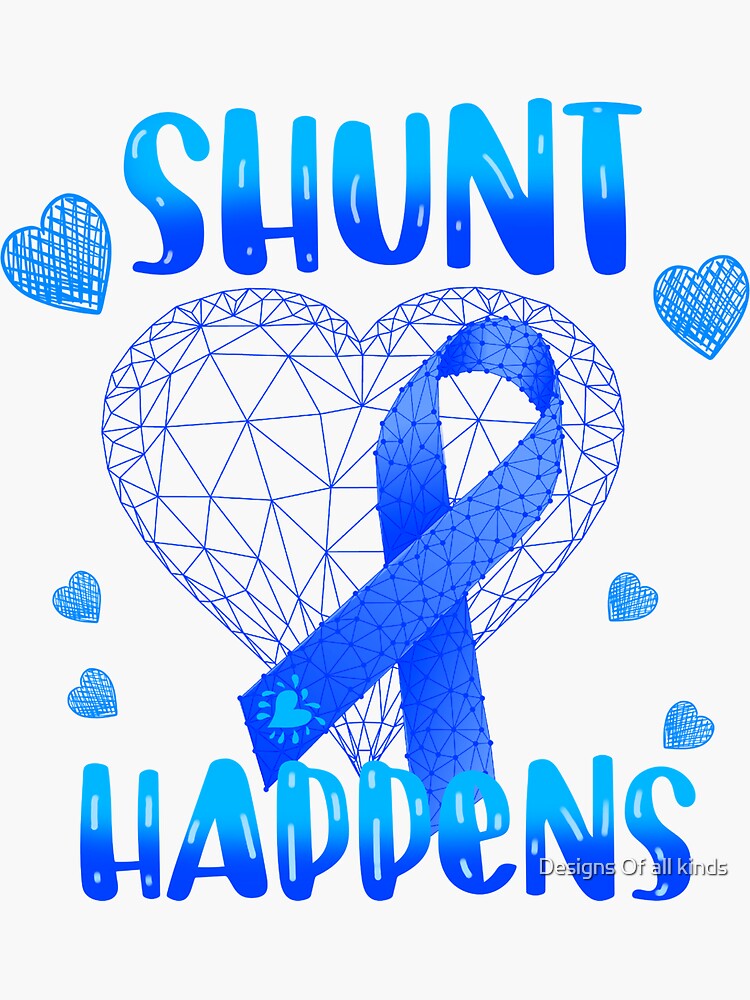The poster features a central geometric wireframe heart in blue, adorned with a large blue ribbon typical of awareness movements, displaying a light blue heart with teardrop motifs on its descending left side. Surrounding this central heart are intricately placed smaller blue hearts—two larger ones at the top and four smaller ones at the bottom, angling toward the center. The title "Shunt Happens" is prominently displayed, transitioning from light blue to dark blue, with "Shunt" above the heart and "Happens" below. The entire composition rests on a pure white background, and the lower right corner bears a watermark that reads "Designs of All Kinds" in white text.